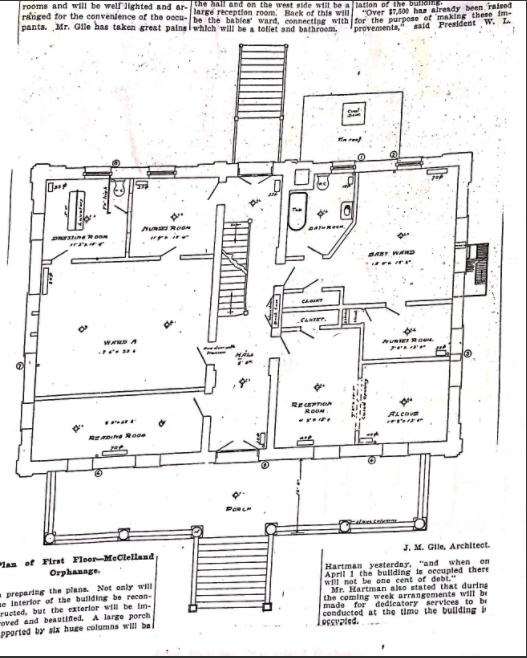This architectural drawing, rendered in detailed black ink on aged white paper, depicts the first floor plan of the McClellan Orphanage, meticulously designed by architect J.M. Guile. The overhead view showcases a layout aimed at convenience and lighting, hinted at by the notes scattered across the page. At the top of the drawing, the text mentions that the rooms are arranged to benefit the occupants. A large reception room on the west side leads to baby wards, connected by a toilet and bathroom. The drawing is framed by two paragraphs at the bottom, providing additional information about the orphanage and its layout. Despite some cut-off writing, the plan reveals multiple rooms, including doors, stairs, closets, and bathrooms, clearly outlined to convey a comprehensive vision of the structure.